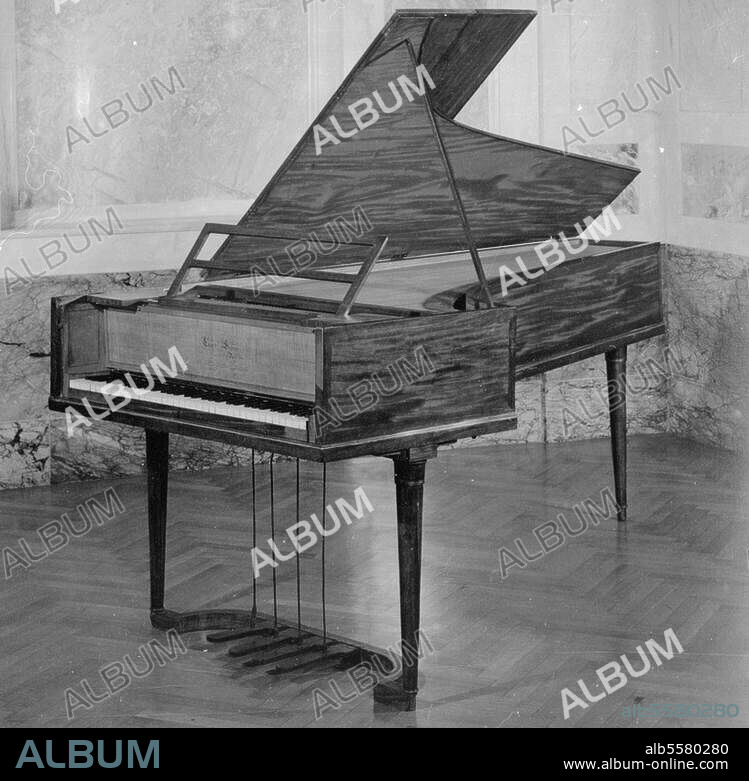The black and white image depicts a grand piano, shown from the right side at a diagonal angle. The piano’s lid is open, revealing the strings inside, and the keyboard is visible without the usual cover, emphasizing an unusual and massive design. Four legs support the instrument, and four foot pedals are visible underneath. Scattered across the picture are watermarks reading "ALBUM" in white and transparent text, deterring any unauthorized use. At the bottom right of the image, a thick black stripe features the text "ALB5580280" and the URL "www.albums.online.com," signifying the image's source and copyright information. The picture has a sketch-like quality, with visible hash lines adding an artistic touch.